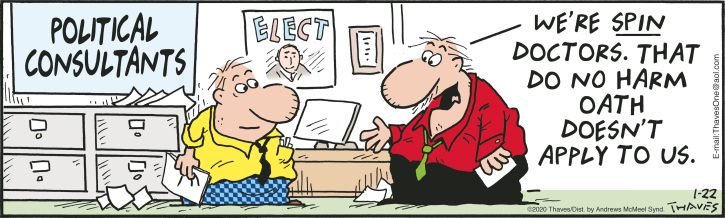This cartoon strip unfolds in an office setting designated by a sign reading "Political Consultants" at the top. The backdrop features a white wall adorned with photo frames and a political poster showing a person and the caption "ELECT." The workspace in the background includes a computer desktop, tables, chairs, and papers strewn across them. The green floor beneath supports two prominent cartoon figures facing each other. Both characters have exaggerated features such as big faces, large noses, and round eyes. The character on the left dons a yellow shirt, black tie, and blue checkered pants, holding a sheet of paper with a pen tucked in his pocket. The right-side character, who appears slightly larger, wears a red shirt, green tie, and black pants, also holding a piece of paper. This character's mouth is open, delivering the bold statement: "We're spin doctors that do no harm, oath doesn't apply to us," with the word "spin" emphatically underlined. At the bottom of the strip, the footnote reads "Copyright 2020, Thaves District by Andreas McMayer-Sin," accompanied by a logo "1 by 22 Thaves" and a vertical email address "Thaves1@AOL.com" in the left corner.